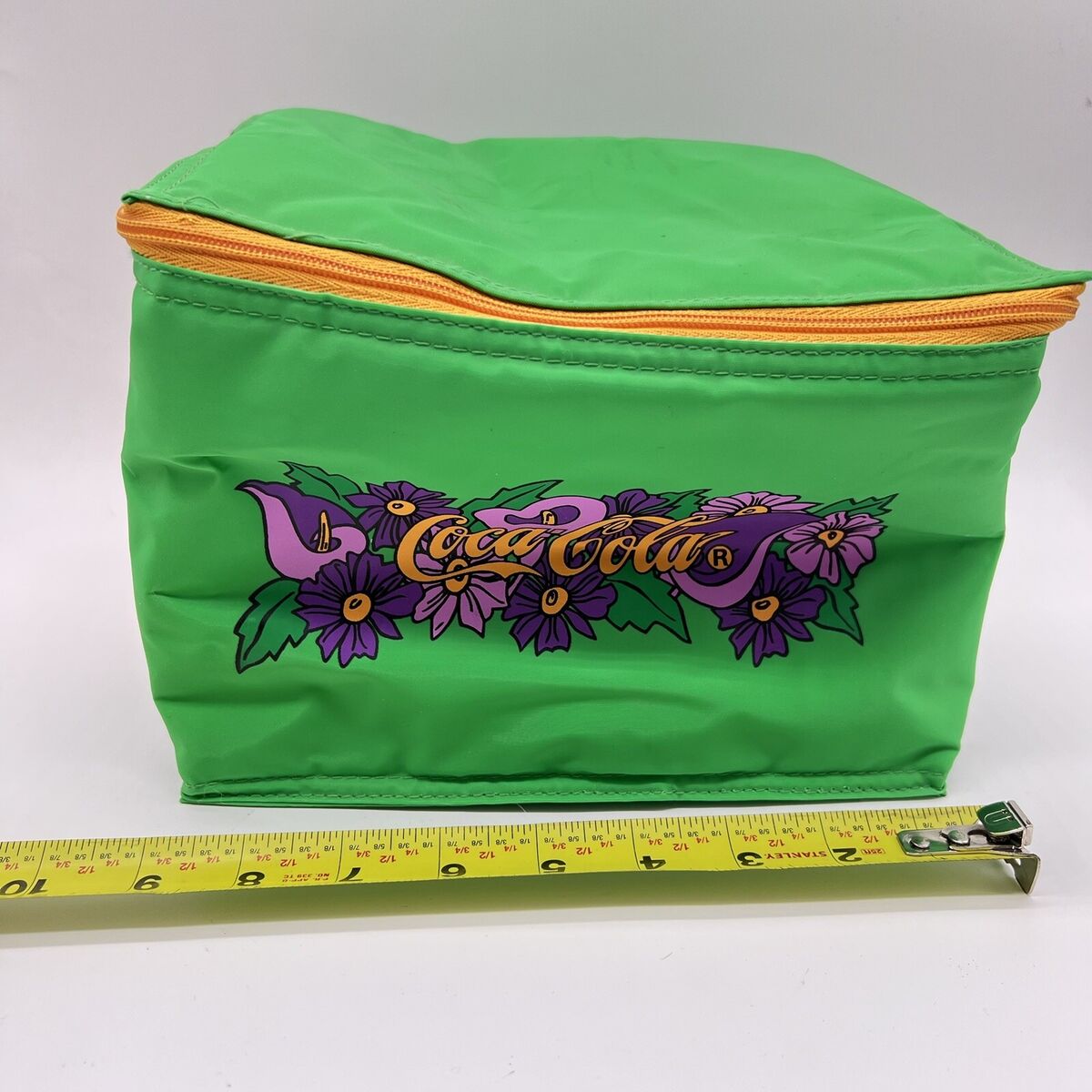The image showcases a compact, foldable cooler crafted from a flexible material. The cooler is predominantly green, accented with a yellow zipper that wraps around its middle. The zipper's yellow lining adds a striking contrast to the overall design. Emblazoned across the front of the cooler, the iconic Coca-Cola logo is depicted in yellow. Surrounding the logo, vibrant purple flowers with yellow centers and green leaves create a lively, eye-catching pattern. Additional purple swirls and more floral designs embellish the area around the logo.

The cooler is positioned against a pristine white background, resting on a white floor. In front of the cooler, a metal ruler lays flat. The ruler, marked with black measurement indicators, is yellow in color and spans up to nine inches. Positioned to measure the width of the cooler, the ruler confirms that the cooler is slightly under nine inches wide.